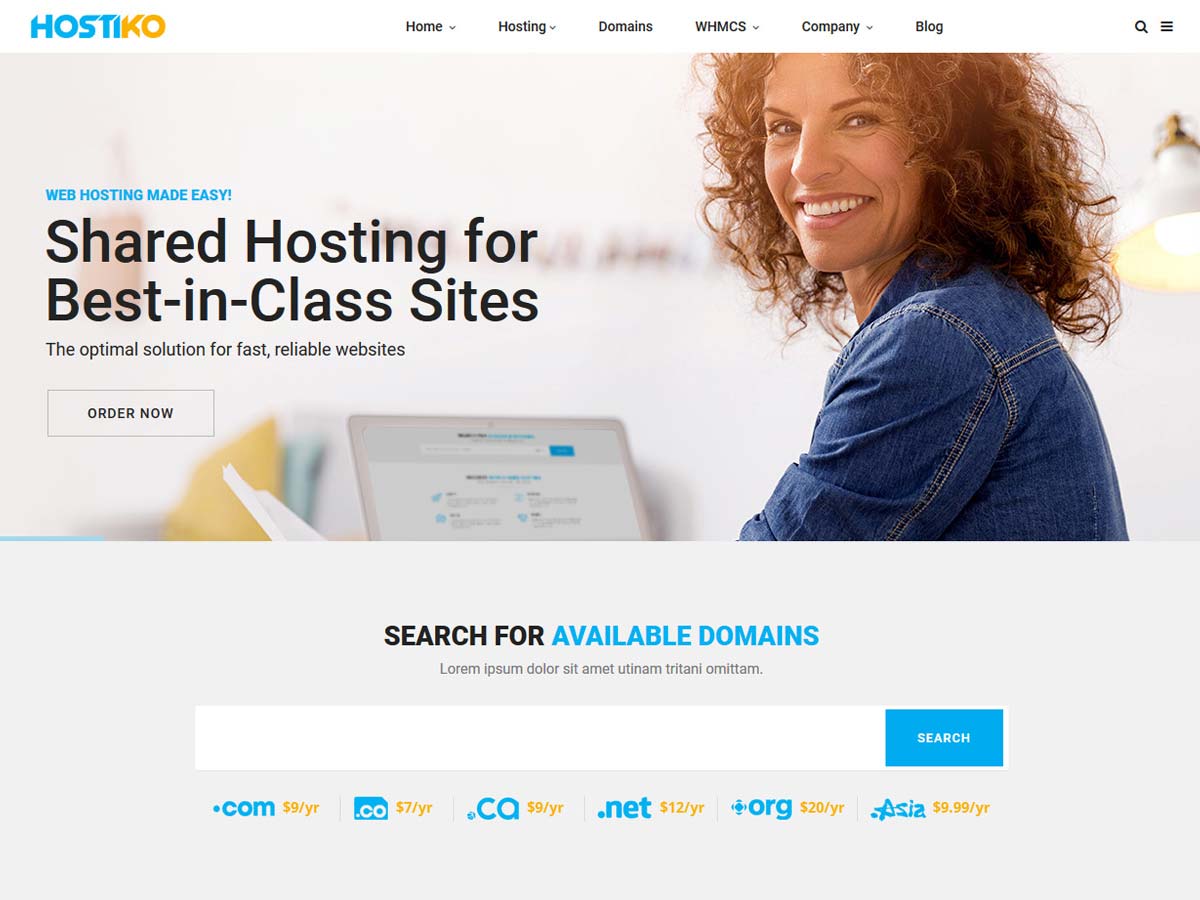Here is a detailed and cleaned-up version of the descriptive caption for the image:

"The image features a webpage from Hostiko, showcasing its web hosting services. At the top, there is a white navigation bar with 'Hostiko' prominently displayed on the left. The text 'HOSTI' is in blue, while 'KO' is in a yellow-orange color. To the right of the logo, the navigation bar includes tabs labeled Home, Hosting, Domains, WHM, CS, Company, and Blog. In the upper right corner, there are a search button and a list button.

Beneath the navigation bar, there is a main visual section featuring a woman with curly brown hair, wearing a blue jean jacket, sitting in front of a laptop. She is smiling and looking back at the camera. To the left of her, the text reads, 'Web Hosting Made Easy: Shared Hosting for Best-In-Class Sites. The Optimal Solution for Fast, Reliable Websites.' Below this descriptive text is an 'Order Now' button.

Further down, the page features a section titled 'Search for Available Domains' with an accompanying search bar, allowing users to look up domain availability easily."